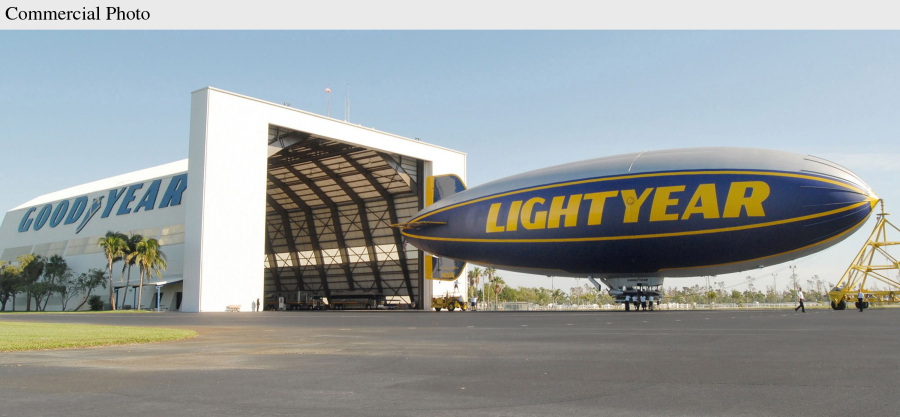In the picture, the iconic Goodyear blimp is being maneuvered out of its large, white hangar that prominently displays the Goodyear name in blue lettering. The blimp itself is blue with yellow stripes and features the word "Lightyear" boldly printed in yellow letters along its side. At the front of the blimp, a tall yellow piece of equipment aids in pulling it out, while at least four people walk nearby, assisting in the process and ensuring its safe exit. The hangar doors stand wide open, revealing a blacktop area stretching out from the entrance. Adjacent to the structure, lush palm trees add a touch of green under a bright, sunny sky. The overall scene is well-lit, accentuated by the clear blue sky, indicating daytime. This appears to be a commercial photo, as mentioned in the gray strip at the top, although this detail doesn’t pertain directly to the visual elements of the image.